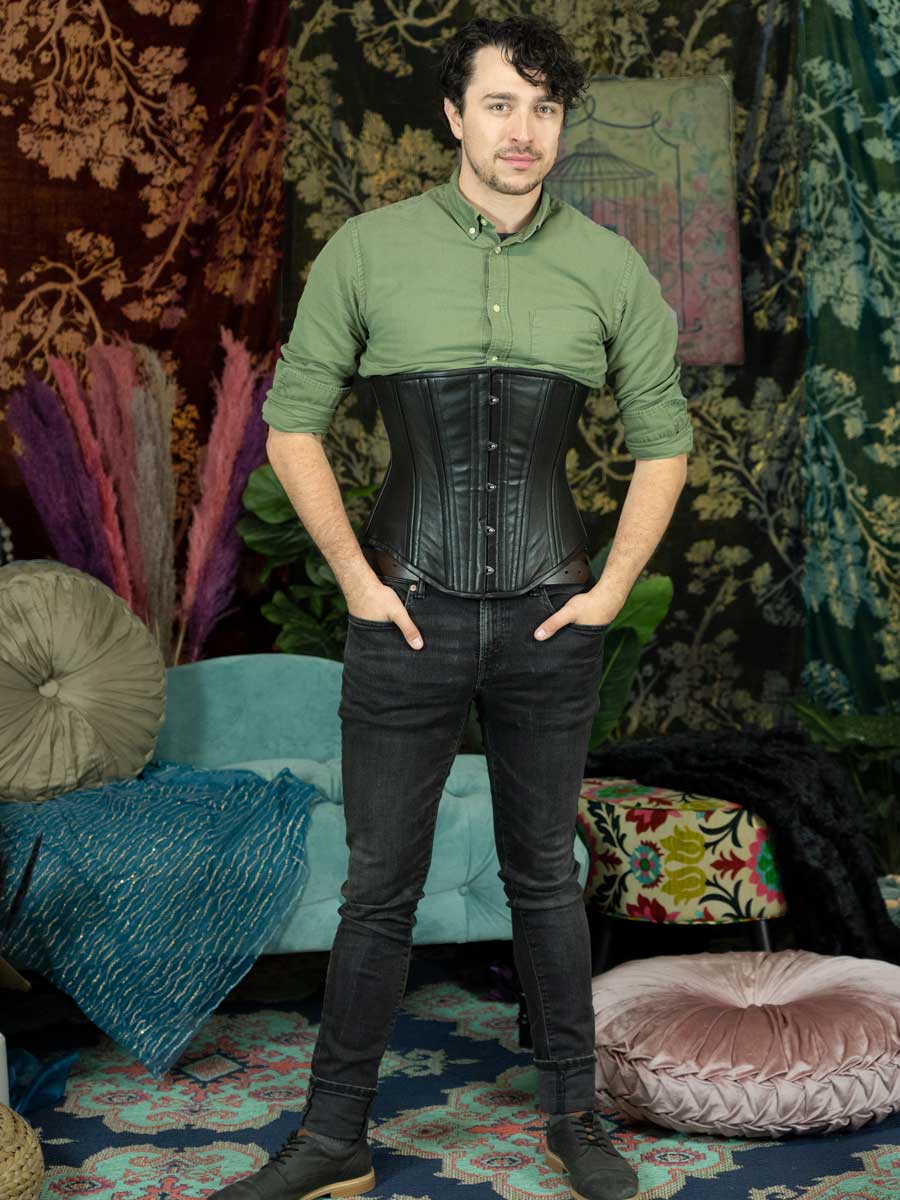The photograph depicts a man, centrally positioned in a highly decorative and colorful room, likely staged for a photo shoot. The man, a white individual with longish, curly brown hair and a slight beard and mustache, is wearing an olive green button-up shirt with its sleeves rolled up to his elbows. Over his shirt, he is modeling a black leather corset. He has black jeans cuffed about two to three inches above the ankle, secured with a brown belt, and wears black shoes with brown soles. His hands rest in his pockets with thumbs protruding.

The background is richly adorned with patterned draperies featuring an array of flowers in golds, blues, oranges, and reds. A teal decorative sofa with a tan circular pillow sits behind him, and additional pillows and blankets are strewn across the floor. There is also a multicolored ottoman, which seems to have a white base adorned with floral patterns in yellows, reds, and blues, and a pink cushion placed on the floor. On the wall hangs an image of an old birdcage, complementing the floral theme with its pink and green hues.

The floor features an ornate blue and teal rug with a repeating pattern in softer shades of blue, pink, light blue, peach, and purple, tying together the colorful and vibrant ambiance of the room. The overall setting is an eclectic and artistic mix of decorative elements, enhancing the photograph's visual appeal.